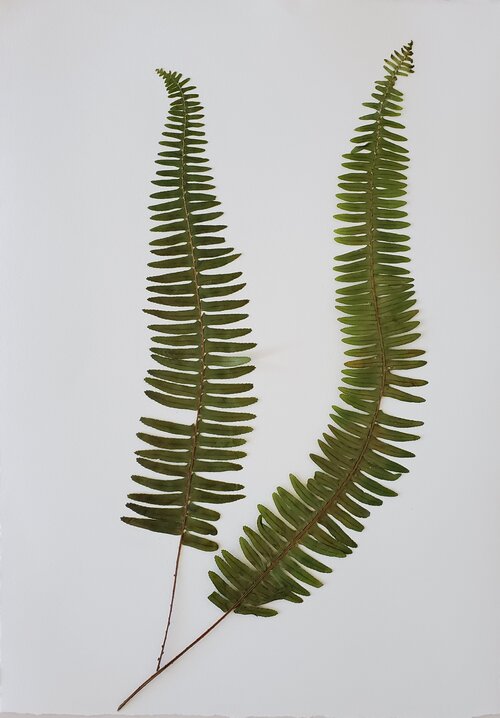Aerial photograph showcasing two elongated stems elegantly arranged on a pristine white background. Each stem, reminiscent of a bone-like structure, stretches vertically from the bottom to the top of the image. Adorning either side of these gracefully extended stems are slender, dark green leaves. The foliage varies in size, with the larger, more pronounced leaves situated at the base, gradually decreasing in size as they ascend towards the top of the stems. The meticulous arrangement and stark contrast between the lush greenery and the clean white backdrop emphasize the delicate beauty and intricate details of the plant life.